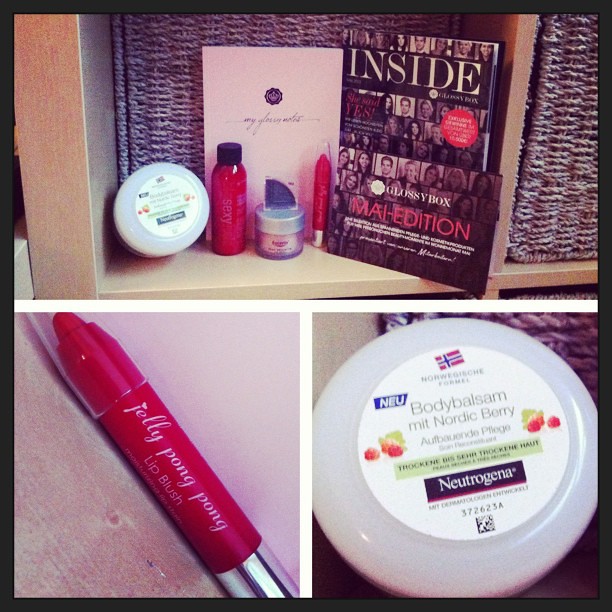The image is a compilation of three photographs, portraying a detailed mail order box of beauty products. The top half, occupying the most space, showcases a display arranged on a shelf with a purple woven background. Central to this display is a magazine titled "Inside" alongside a card labeled "Glossy Box Mail Edition". Surrounding these are various beauty products, including a prominent red cylindrical tube labeled "Jelly Pong Pong Lip Blush", a round container with the Norwegian flag labeled "Body Balsam Mint Nordic Berry" by Neutrogena, and other smaller cosmetic items. These items seem to include a red cylindrical bottle with a blue cap labeled "Sexy", and a small pink jar. The bottom of the image is split into two close-ups: the left highlights the "Jelly Pong Pong Lip Blush" tube in greater detail, while the right magnifies the "Body Balsam Mint Nordic Berry" container from Neutrogena, showcasing its branding and berry illustrations. Together, these photos intricately present a curated selection of beauty products from a Glossy Box mail edition.